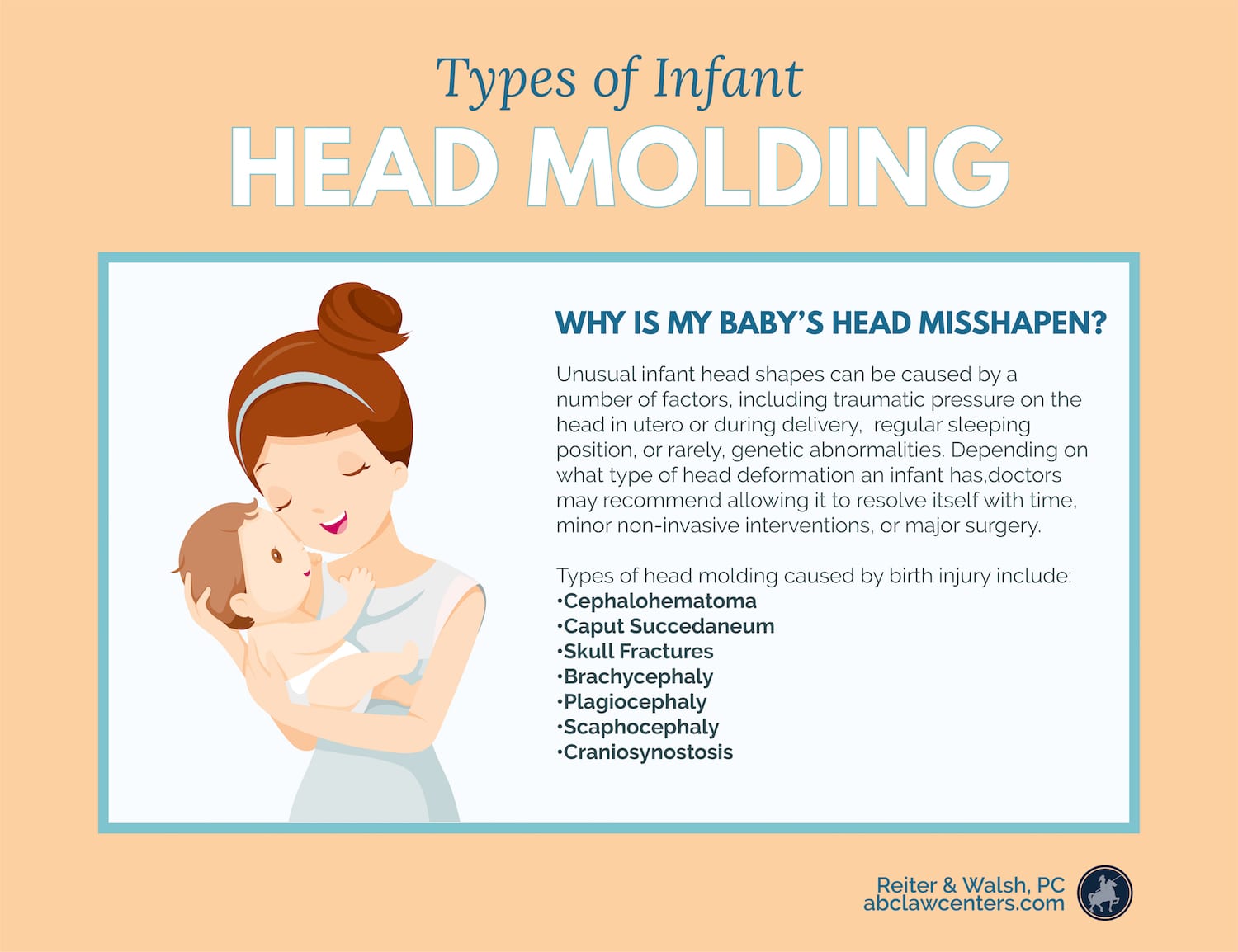This graphic, presented on a pinkish-tan background, serves as a public service announcement regarding infant head molding. Titled "Types of Infant Head Molding" in bold blue and white text at the top, it aims to address parental concerns with the subtitle, "Why is my baby's head misshapen?" It explains that unusual infant head shapes can result from factors such as traumatic pressure during pregnancy or delivery, consistent sleeping positions, or genetic abnormalities. Depending on the type of head deformation, doctors might recommend various interventions ranging from allowing the condition to resolve naturally to considering major surgery. The visual features a smiling mother with brown hair in a bun, a blue headband, and a white bluish dress, holding her smiling baby in diapers, who has light brown hair and is looking up at her with admiration. The entire background is light yellow, and the bottom right contains the attribution to the law firm, "Reiter & Walsh, P.C.", with the website "abclawcenters.com" alongside a logo depicting a stamp with a person on a horse.